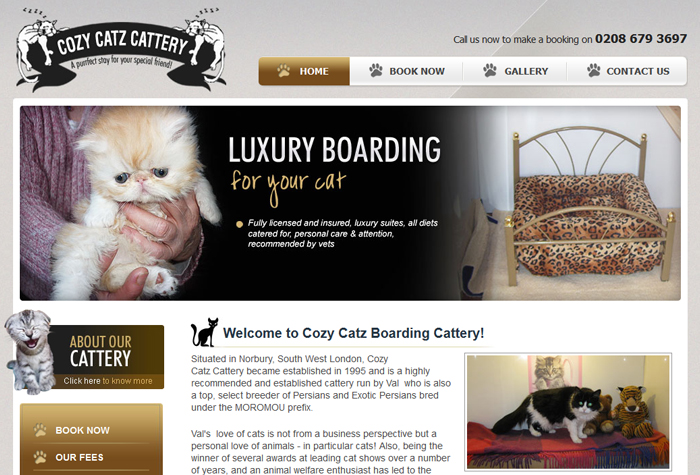Screenshot of the Cozy Cats Cattery Website

The image is a rectangular screenshot of a website dedicated to boarding pet cats. The background is primarily gray. In the top right corner, there's a logo consisting of a black banner with white text reading "Cozy Cats Cattery," and beneath it, a subtitle in black text, "A Perfect Stay for Your Friend." Flanking the banner are two illustrations of white sleeping cats. 

Positioned below the logo is a horizontal menu with four selectable boxes. The leftmost box is brown with white text reading "Home." The three remaining boxes are white with black text, labeled "Book Now," "Gallery," and "Contact Us." Above this menu, black text announces, "Call Us Now to Make a Booking on 0208-679-3697."

The main body of the webpage features a white rectangular background. At the top of this area, there's a large banner. On the left side of the banner, an individual is seen holding an orange and white cat with both hands. In the center of the banner, white and orange text reads, "Luxury Boarding for your cat."

This descriptive caption captures the layout and contents of the Cozy Cats Cattery website screenshot in detail.